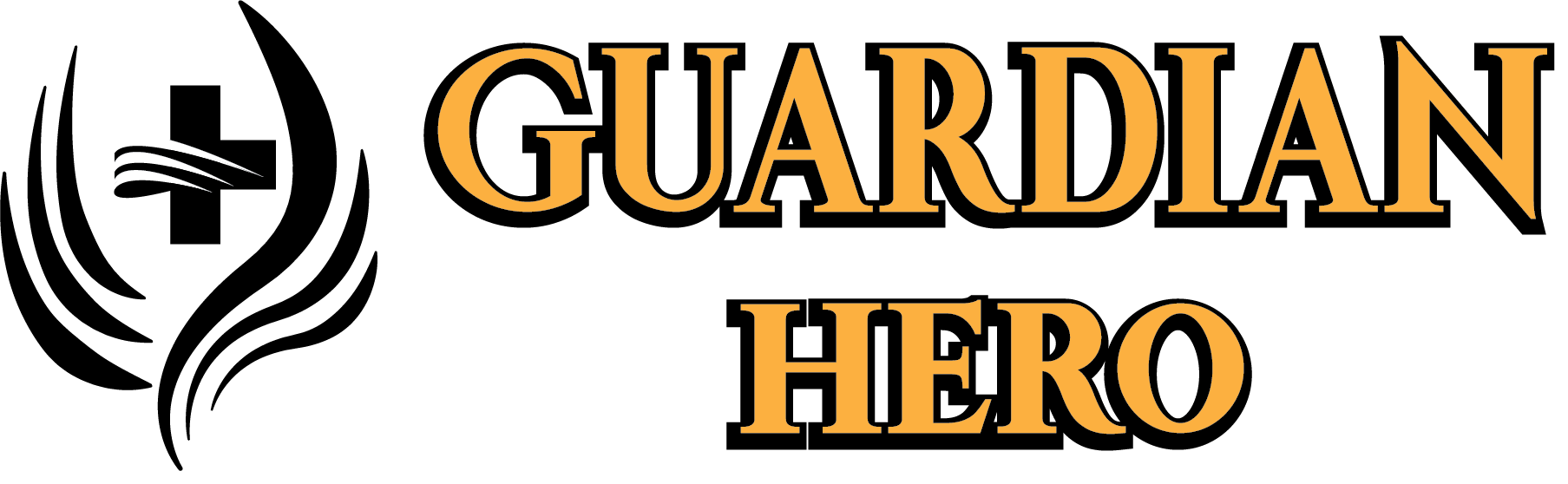The image prominently displays the words "GUARDIAN HERO" in a bold, all-caps Times New Roman-like font. The text is mustard orange with a black outline, creating a shadowed effect. "GUARDIAN" is positioned above "HERO," making the words stack neatly. To the left of this text is a black and white emblem. Central to the emblem is a black plus sign, which may be interpreted as a cross. On the left side of the plus sign, three white, thick, curved lines, resembling stylized hairs or swirls, extend and taper into points. These lines cover the left arm of the plus and are arranged in a slightly staggered pattern. Surrounding the plus sign, there are also three matching black curved figures on both the left and right sides. On the left, these black shapes are reminiscent of the left side of parentheses, stacked but not touching, with each consecutive figure positioned slightly lower and thicker than the previous one. On the right, three black curvy lines -- the closest one being thicker and more pronounced -- mirror the left shapes, curving around the plus sign as if beginning to form an 'S' but stopping short. The overall effect is a cohesive and well-balanced design, pairing bold text with an intricate, symbolic emblem.